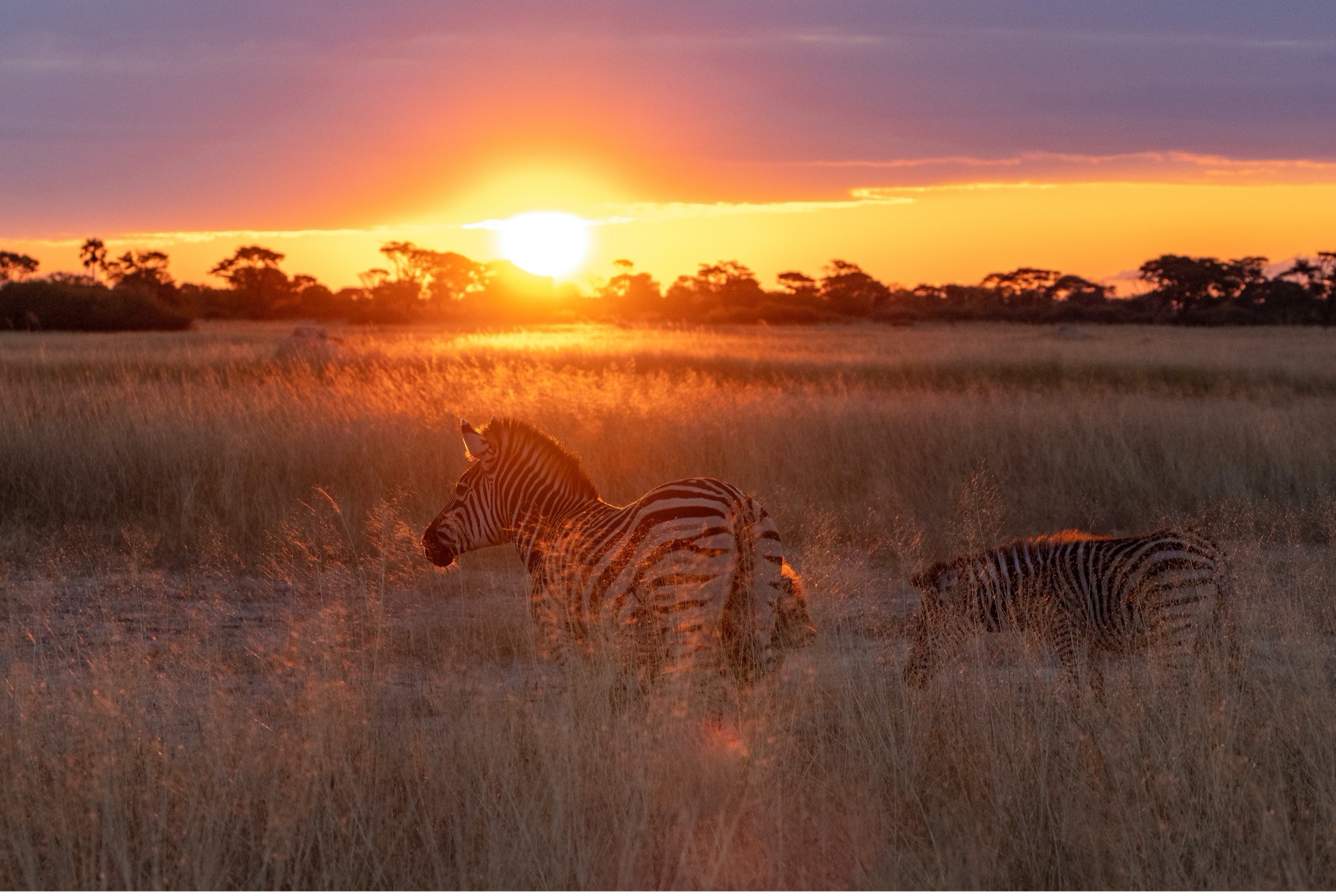The image captures a striking scene of the savannah at sunset, showcasing two zebras in the foreground. The sky is a blend of light blue, orange, and white hues, as the sun sets behind a horizon adorned with low-lying trees, characteristic of the African plains or Serengeti. The entire horizon is silhouetted, with purple clouds stretching across the upper portion of the sky, creating a vivid yet serene backdrop.

In the foreground, two zebras with distinct black and white stripes are seen grazing amid tall, beige grass. The closest zebra, slightly left of center, stands with its head up, partially turned to the left, and appears larger, likely indicating it is nearer to the camera. The second zebra, positioned to the right and a bit farther away, has its head bent down, possibly grazing, and is partially obscured by the grass.

The overall composition of the photograph, with its realistic and representational style, beautifully captures the essence of the savannah landscape and the quiet elegance of the zebras within their natural habitat.